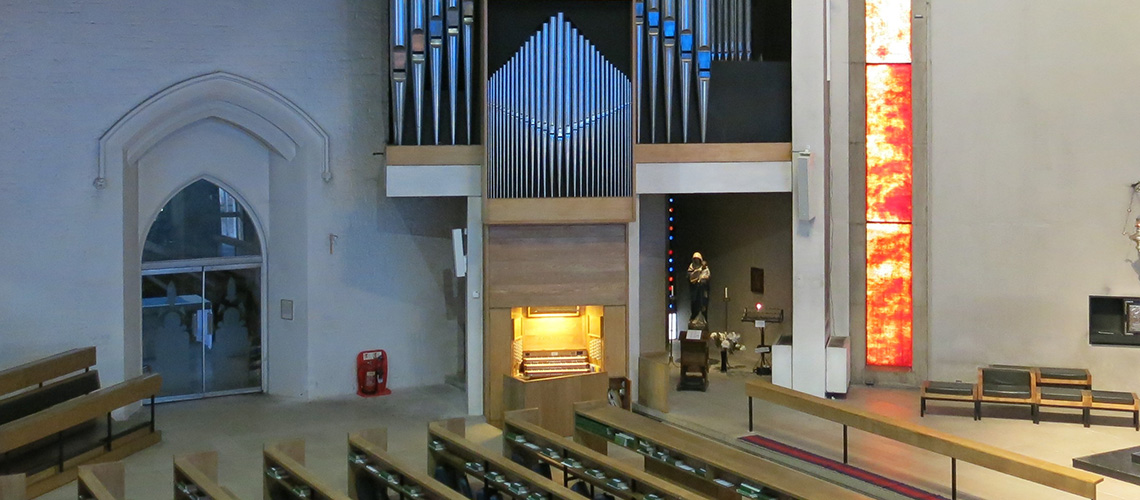The image portrays a spacious and well-lit church interior. Dominating the center of the composition is a luminous enclave housing a pipe organ, identifiable by the array of pipes that soar upward and converge to a point above it. This organ space, framed with light wood, is bathed in natural light that accentuates its presence. To its immediate right, a vibrant red-orange stained glass window casts colorful reflections, enhancing the serene atmosphere. Adjacent to this window, a simple wooden bench rests quietly. On the left side of the organ, a glass doorway crowned by an arched window allows additional light to filter through. In the lower portion of the image, rows of empty pews stretch from the foreground toward the back wall, which is painted a light gray. The upper right quadrant also contains a secondary enclave that features a statue, possibly of the Virgin Mary, accompanied by an altar and podium, creating a solemn spot for prayer and reflection. The overall color palette includes shades of white, brown, tan, blue, yellow, and red, contributing to the church's warm and inviting atmosphere. The setting suggests daytime, with a sense of tranquility prevailing in the empty, sacred space.